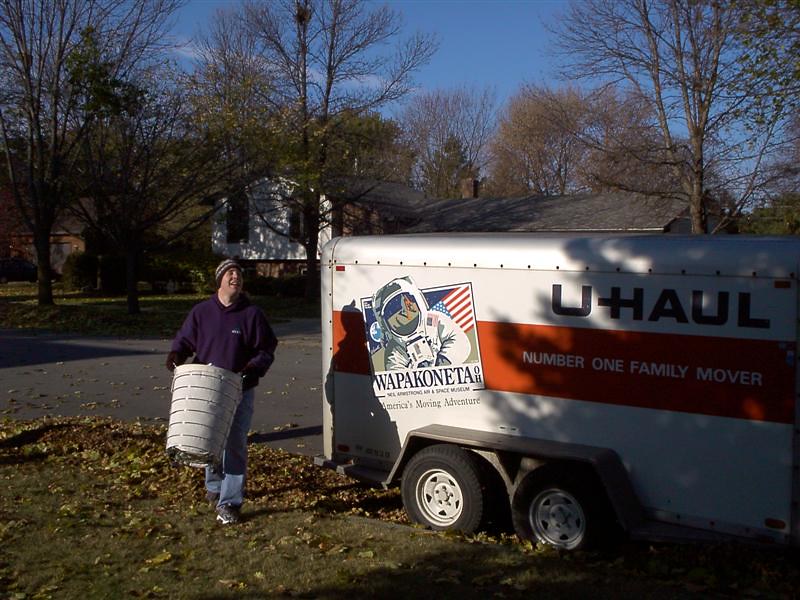A white U-Haul van with an orange horizontal section in the middle is parked by the curb, prominently displaying "number one family mover" on its side. Near the rear of the van, there's an illustration of an astronaut named Armstrong planting a U.S. flag. Standing to the left of the van, a man dressed in a purple long-sleeved top, blue jeans, a coat, and a hat holds a white bucket, seemingly about to place it in the van. The backdrop features houses with typical tile roofs and some trees across the street, whose foliage appears mostly gone. The area has leaves scattered on the ground, suggesting a scene in late autumn. The skyline beyond the trees looks clear, contributing to a serene suburban setting.